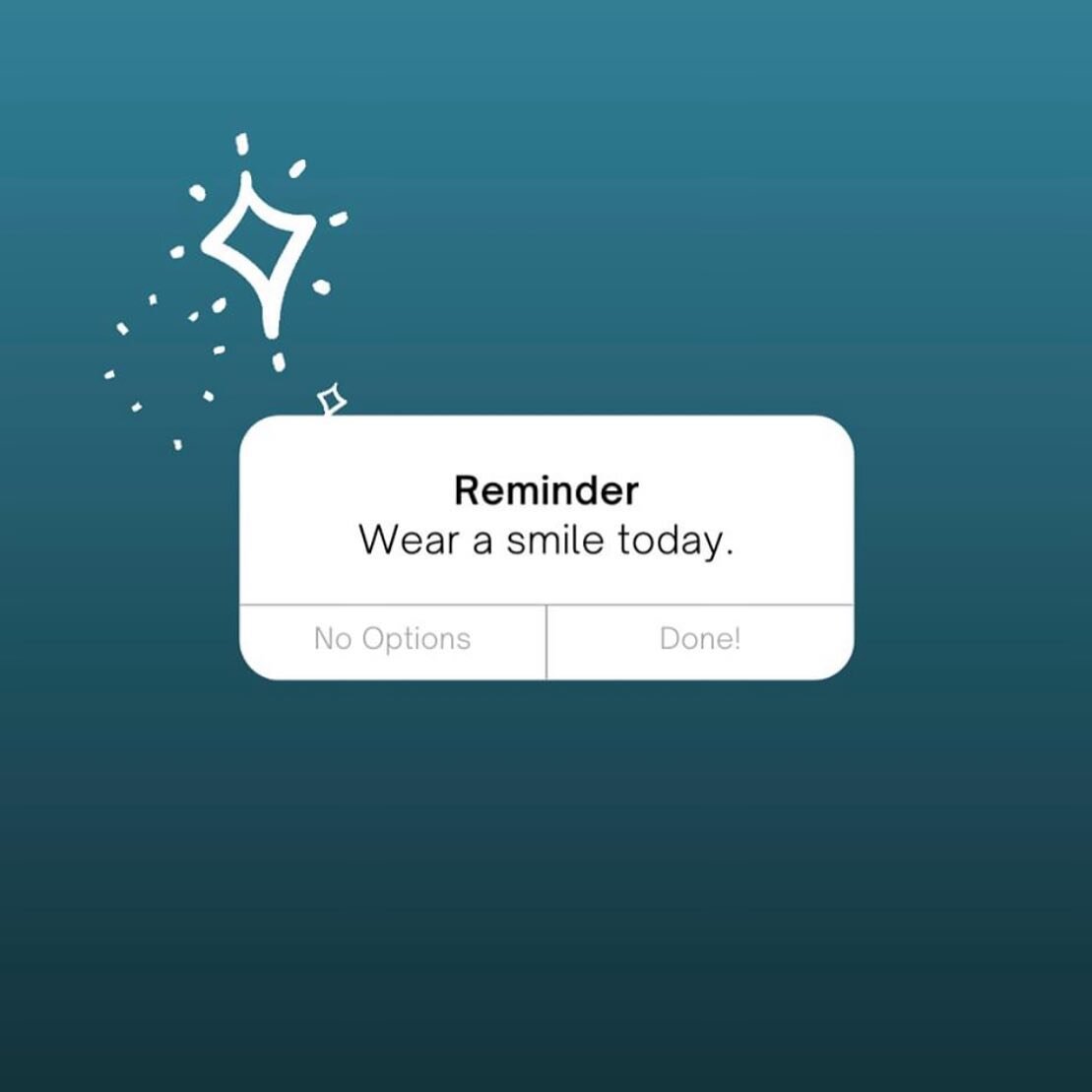The image on the computer screen features a gradient background transitioning from a dark blue-black at the bottom to a lighter blue at the top. In the center of the image, there is a rounded rectangle with a darker black border containing two sections of text. The first section reads "Reminder" in bold black font. Directly below this, in lighter print, is the phrase "Wear a Smile Today." Underneath these texts, a thin light gray line separates the sections. Below this line are two interactive boxes; one labeled "No Options" and the other labeled "Done!" with an exclamation point. 

Within the "Done!" box, there is a stylized illustration resembling a light bulb but shaped like a diamond, rendered in thick white lines. Surrounding the diamond are radiating lines suggesting rays of sunshine. To the right of this illustration, a series of ray-like lines form a circle, without a solid colored center. Additionally, a small diamond-shaped object is positioned near the top of the box, adding a subtle decorative element to the otherwise minimalist design.